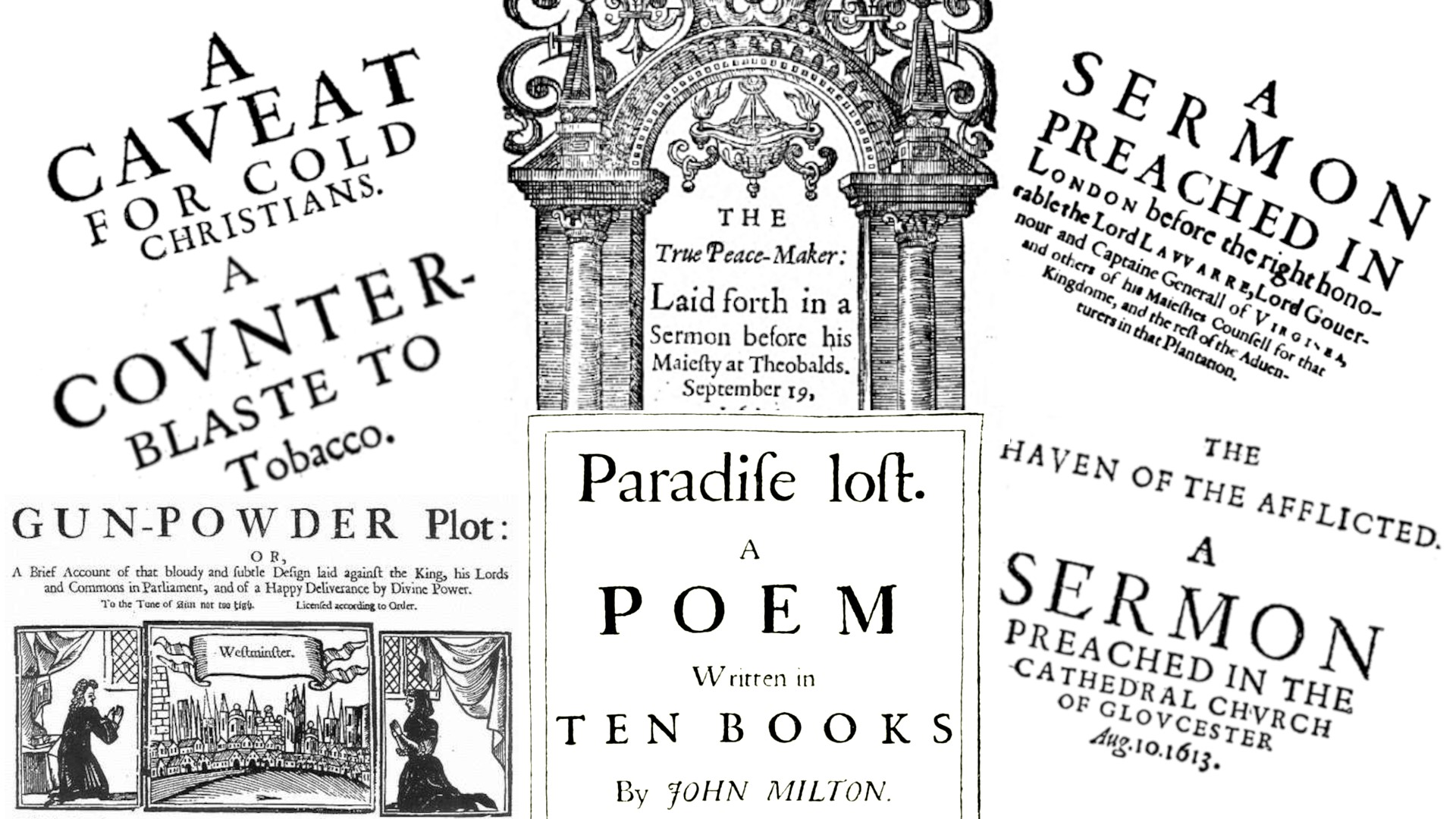This image is a black-and-white collage of vintage book title plates and frontispieces, each showcasing intricate details and historical texts. Central to the composition is an ornate archway, meticulously carved and featuring a chandelier hanging in the center. The archway encloses the title, "The True Peacemaker, Laid Forth in A Sermon Before His Majesty at Theobald's, September 19th." Below this, framed in a rectangle, are the words "Paradise Lost, A Poem Written in Ten Books by John Milton," featuring old-style typography where 's' appears as 'f'.

On the left side, several titles are listed: "A Caveat for Cold Christians" and "A Counterblast to Tobacco." Below these, "Gunpowder Plot" appears, accompanied by a detailed three-panel illustration depicting two people praying on either side of an engraving of Westminster Abbey. 

On the right side, more titles are presented: "A Sermon Preached in London Before the Right Honourable the Lord Le Var, Lord Gouverneur, and Captain-General of Virginia," followed by "The Haven of the Afflicted: A Sermon Preached in the Cathedral Church of Gloucester, August 10th, 1613." All text is rendered in old-timey fonts, enhancing the vintage aesthetic of the piece.